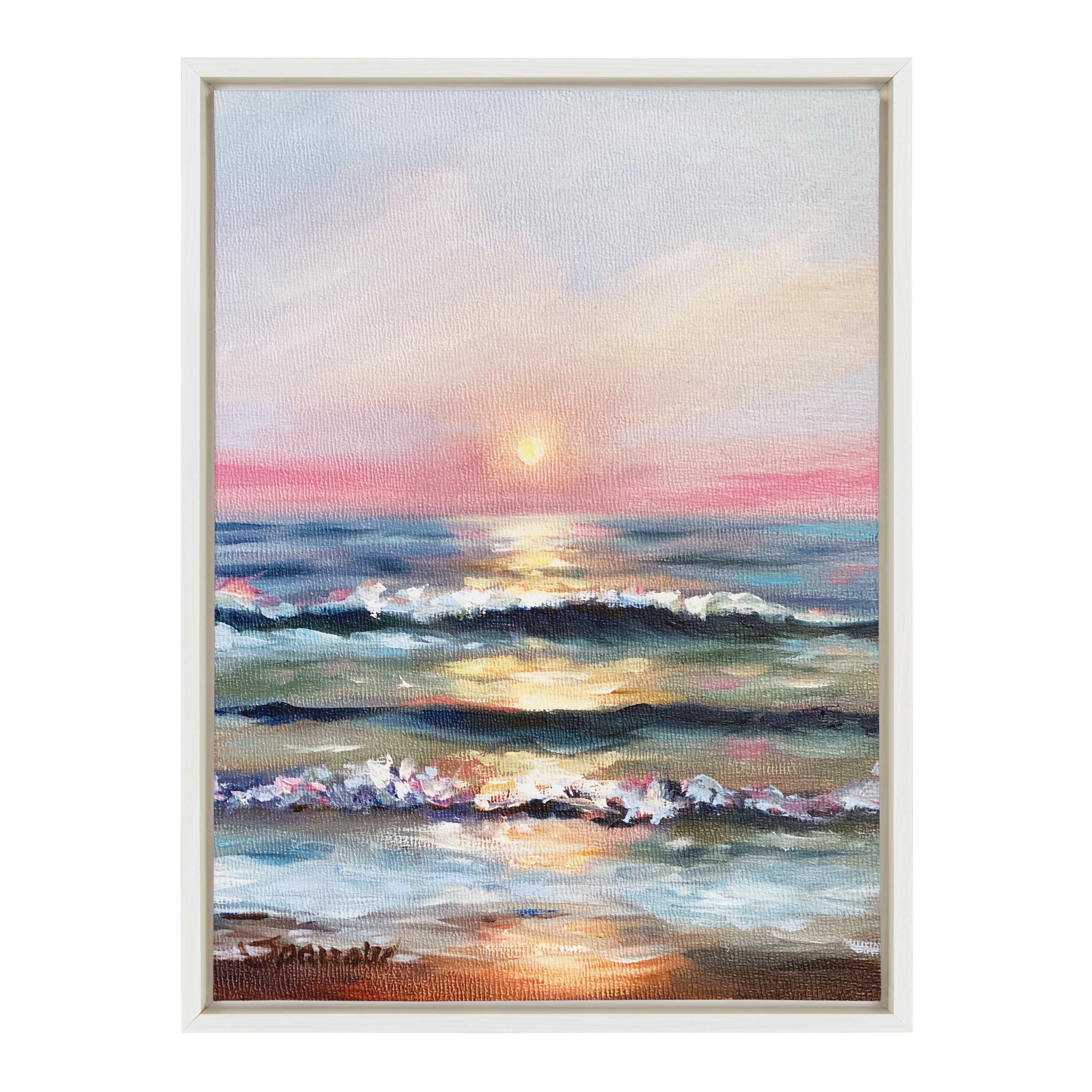The painting captures a stunning sunset over an expansive ocean horizon. It is a rectangular watercolor piece, framed with a thin white border and accented by a wider gold one, with gold writing complementing the frame. The sky transitions from a deep blue at the top, to a light yellow, and then a warm pink near the sea level. At the center of this gradient, the yellow sun is depicted setting over the ocean, casting a vivid, bright yellow reflection across the water. The sea mirrors this colorful palette, blending from blue near the horizon to greenish-yellow and then light blue closer to the shore. The water features gentle waves with white crests, idly lapping at the shore, which is rendered in an orangey-yellow and brown tint. To the left side of the shore, there's an artist's signature, though it is not legible. The entire scene evokes the serene and picturesque beauty of a beach at sunset.